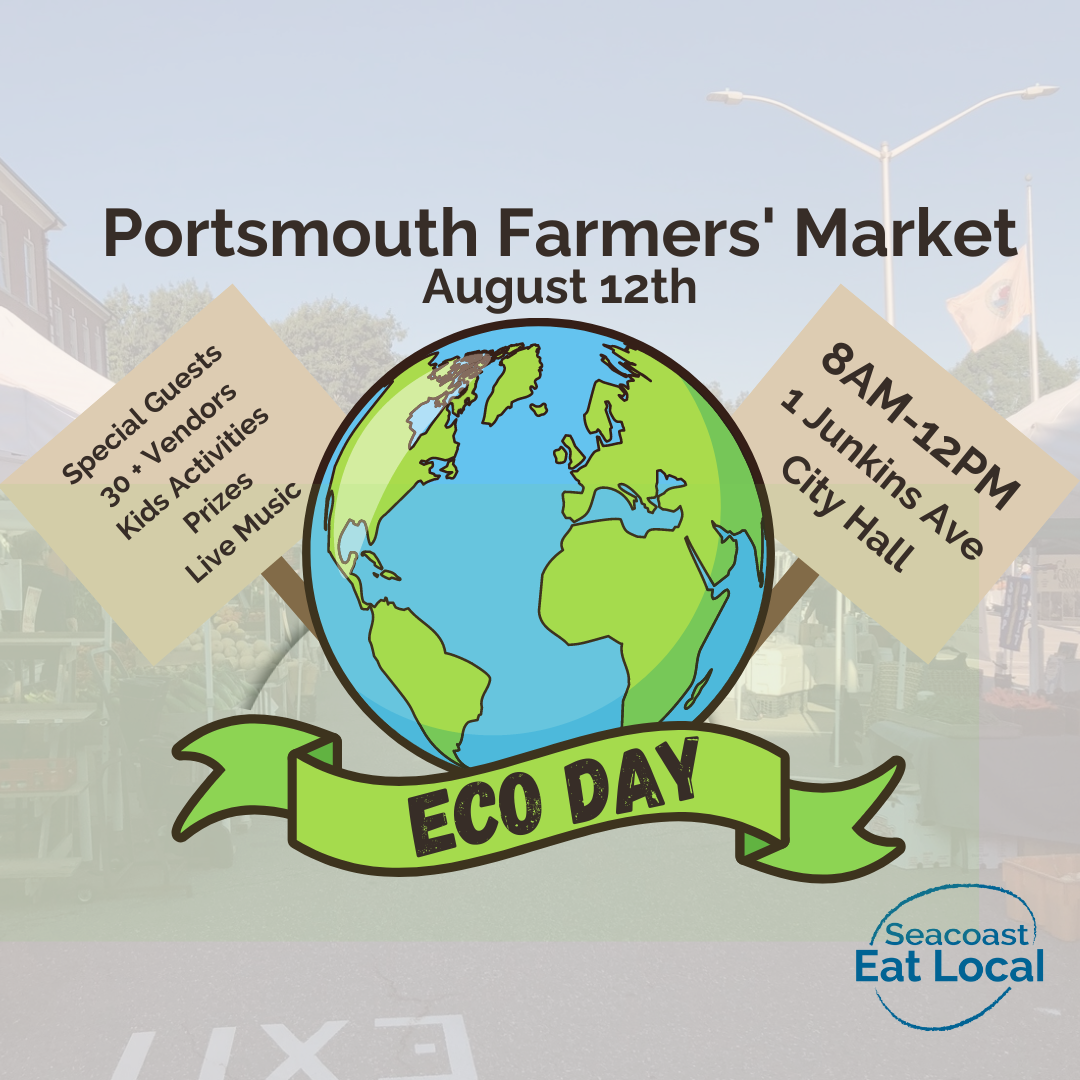The image is a vibrant and detailed poster advertising the Portsmouth Farmers Market scheduled for August 12th. At the top, the text "Portsmouth Farmers Market, August 12th" is prominently displayed. The centerpiece of the poster is a large, cartoonish depiction of the globe, vividly showcasing the continents in green and the oceans in blue. Below the globe, a green banner inscribed with "Eco Day" highlights the event's environmental theme.

On either side of the globe, beige signs with black writing provide additional details: the left sign lists "Special Guests, 30+ Vendors, Kids Activities, Prizes, and Live Music," while the right sign notes the time and location: "8 a.m. to 12 p.m., 1 Junkins Avenue, City Hall."

A faded background image of an open-air market scene fills the whole poster, depicting white tents, flags, buildings, and streetlights, suggesting the lively ambiance of a bustling street market closed off to accommodate various vendors. At the bottom of the poster, an emblem in blue font reads "Seacoast Eat Local," reinforcing the community-focused and local initiative aspect of the event.